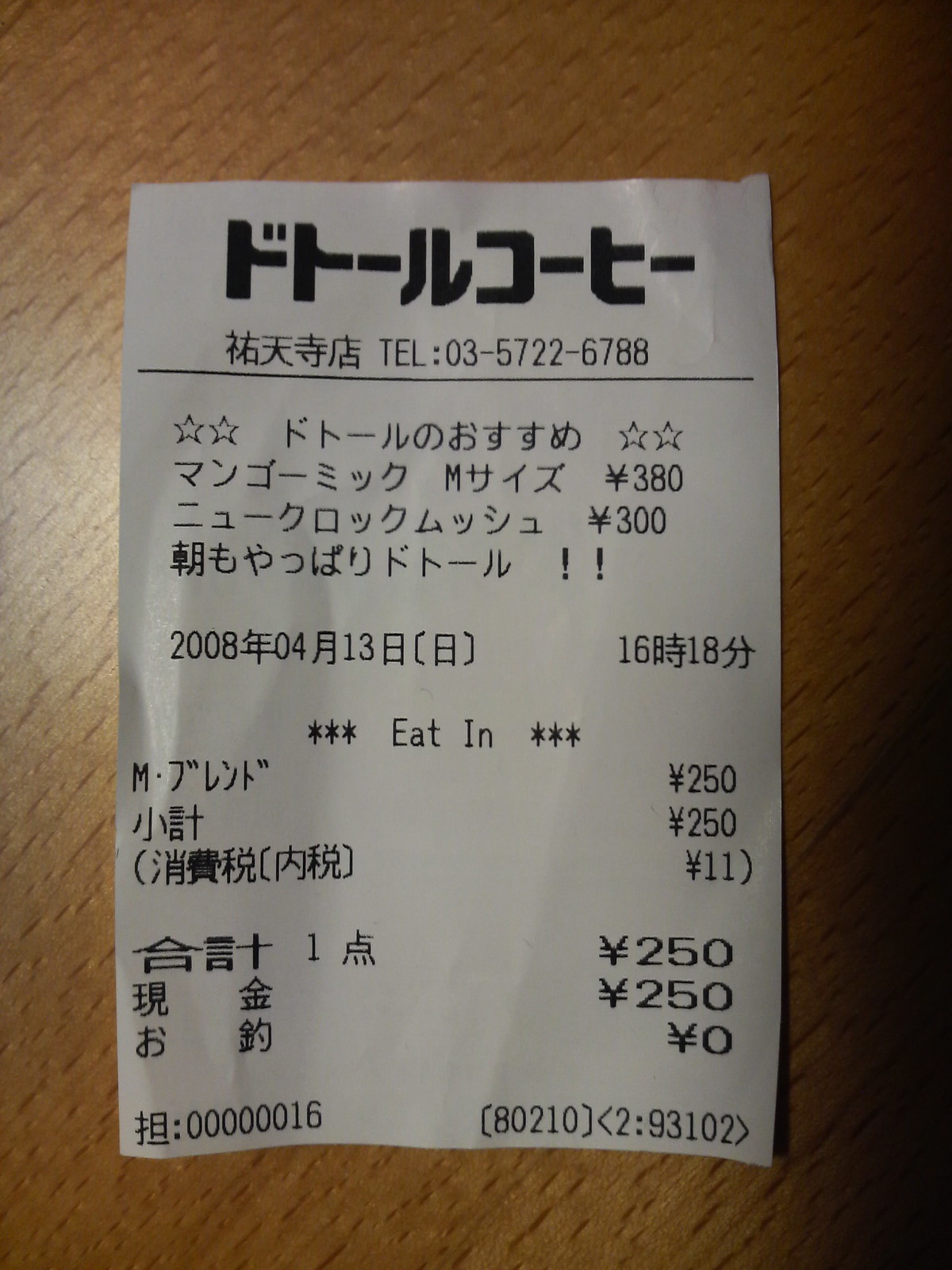The image shows a receipt from a foreign country, possibly Japan, as indicated by the prominent use of Asian script and the appearance of the yen symbol (¥). At the top of the receipt, there is bold lettering followed by a line of text with characters that may suggest Japanese origin. Below this text, the receipt features two stars on one side, followed by additional information, then two more stars, and subsequent details. The numbers "380" and "2008" are visible, and the date "2008-04" suggests the receipt's issuance date. The total amount listed is 250 yen, and at the very bottom, there appear to be several serial numbers or identification codes.